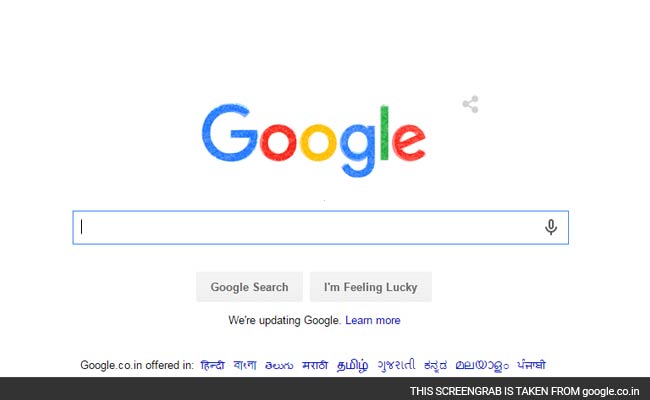A screenshot of the Google homepage (google.com.co.in) captured from a computer screen. The familiar Google logo appears in color prominently at the center of the page. Below the logo, there's a search bar where users can input their queries. Beneath the search bar, there are two clickable buttons: "Google Search" and "I'm Feeling Lucky." Below these buttons, there is a notice stating, "We're updating Google," with a "Learn more" link in blue font. Towards the bottom of the image, just above the black bar indicating the regional site in use, it displays “Google.co.in offered in” followed by a list of nine clickable languages, each displayed in a blue font. This comprehensive layout underscores Google’s multilingual support and user-friendly design for the Indian market.